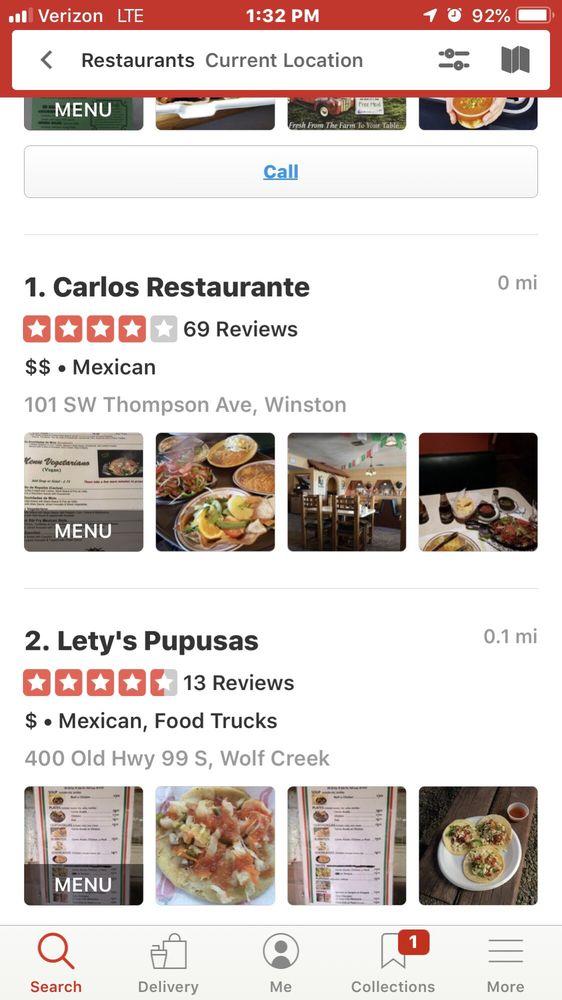A screenshot of a web page listing various restaurants near the user's current location. At the top of the page, there's a navigation bar titled "Restaurants Current Location." Directly below, a blue, underlined "Call" option is presented. The first restaurant listed is "Carlos Restaurante," marked as number one. This establishment is listed as being zero miles away, boasts a rating of four out of five stars based on 69 reviews, and is categorized with two dollar signs, indicating moderate pricing, followed by a dot and the label "Mexican." 

The restaurant's address is provided in lighter-colored text: "101 Southwest Thompson Avenue, Winston." Below this textual information are four small image thumbnails arranged horizontally. The first thumbnail gives a small, unreadable glimpse of the menu. The second thumbnail shows a dish that includes lemon wedges, presenting an appetizing look. The third thumbnail features an interior shot of the restaurant, highlighting wooden chairs. The fourth thumbnail displays a table set elegantly with white linens and silverware.